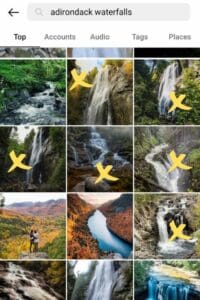The image depicts a search engine results page where the query "Adirondack Waterfalls" has been entered into a gray search bar at the top. Below the search bar, a series of categorized tabs are visible, including options such as "Top," "Accounts," "Audio," "Tags," and "Places." Displayed prominently are 12 thumbnail images related to the search, though only nine of these images are fully visible, with a few being partially cut off.

The majority of these images feature stunning waterfalls, varying in size and height—from towering falls that seem to plummet several hundred feet, to shorter, more compact cascades. Six of these images are marked with a yellow 'X,' a detail whose significance is unclear. It might indicate the user's favourites or images they intend to discard.

Among the waterfall images, one stands out as it depicts a man and a woman with no visible waterfall in the background, distinguishing it from the others which predominantly capture the natural beauty of the Adirondack waterfalls. The photos collectively showcase an array of picturesque waterfalls, highlighting the diverse and breathtaking scenery of the Adirondacks.